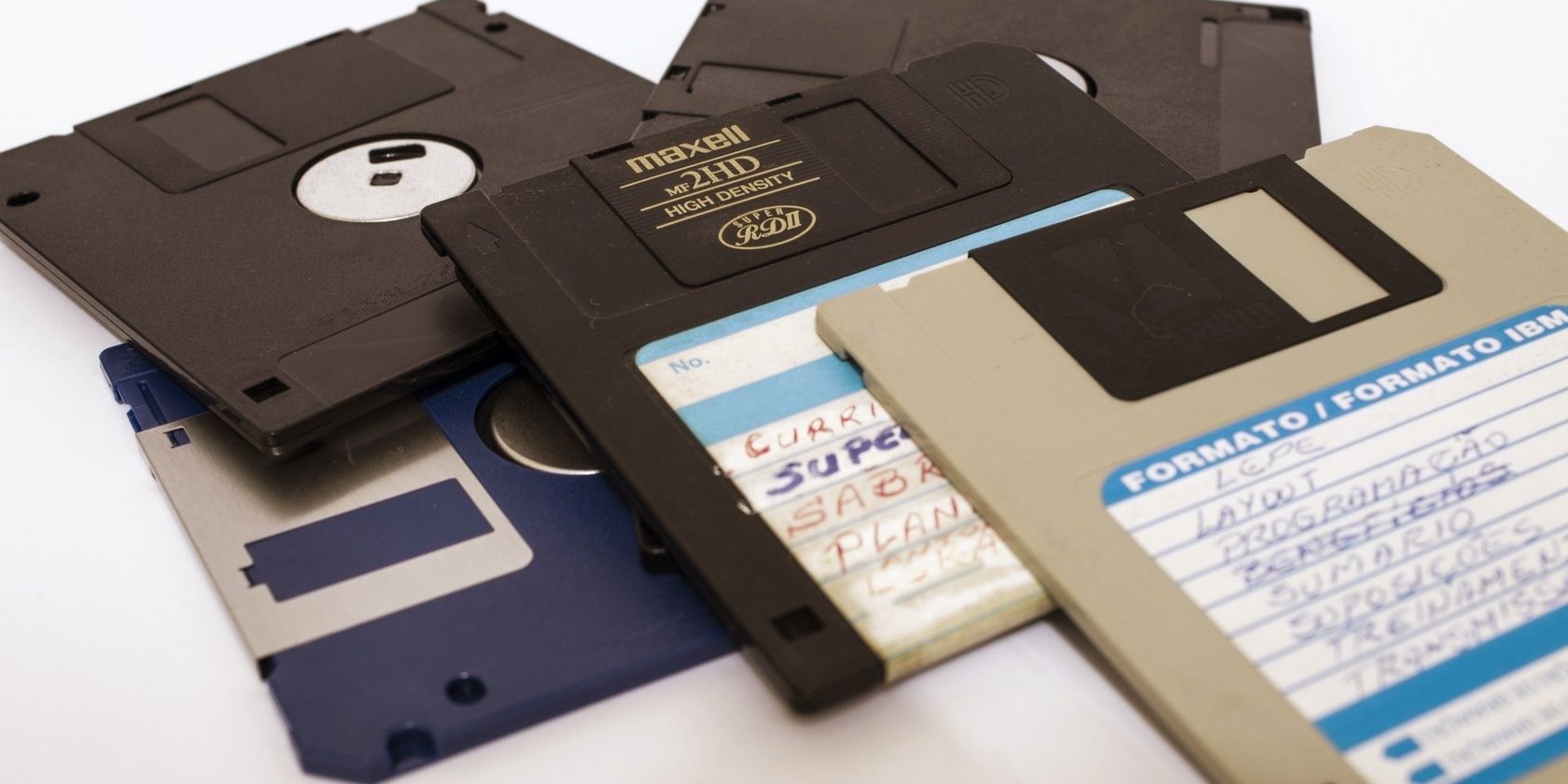The image showcases a close-up, staged photograph featuring an assortment of old floppy disks arranged in a landscape style on a white table. There are five disks in total, predominantly in shades of black and gray, with one distinctive purple disk adding a splash of color. Among the disks, various handwritten labels are visible, mostly written in blue pen and marker, although the specific details are hard to decipher. Words like "layout," "programming," and "Formato IBM" can be seen on the labels in both English and Spanish. The disks include those branded Maxell MF2HD High Density, identifiable by their gold font on a darker black disk. The floppy disks are arranged in a single layer: a navy blue and white disk at the bottom, followed by two matte black disks, then a darker black disk with a gold-font label, and a tan disk with a blue and white striped label on top.